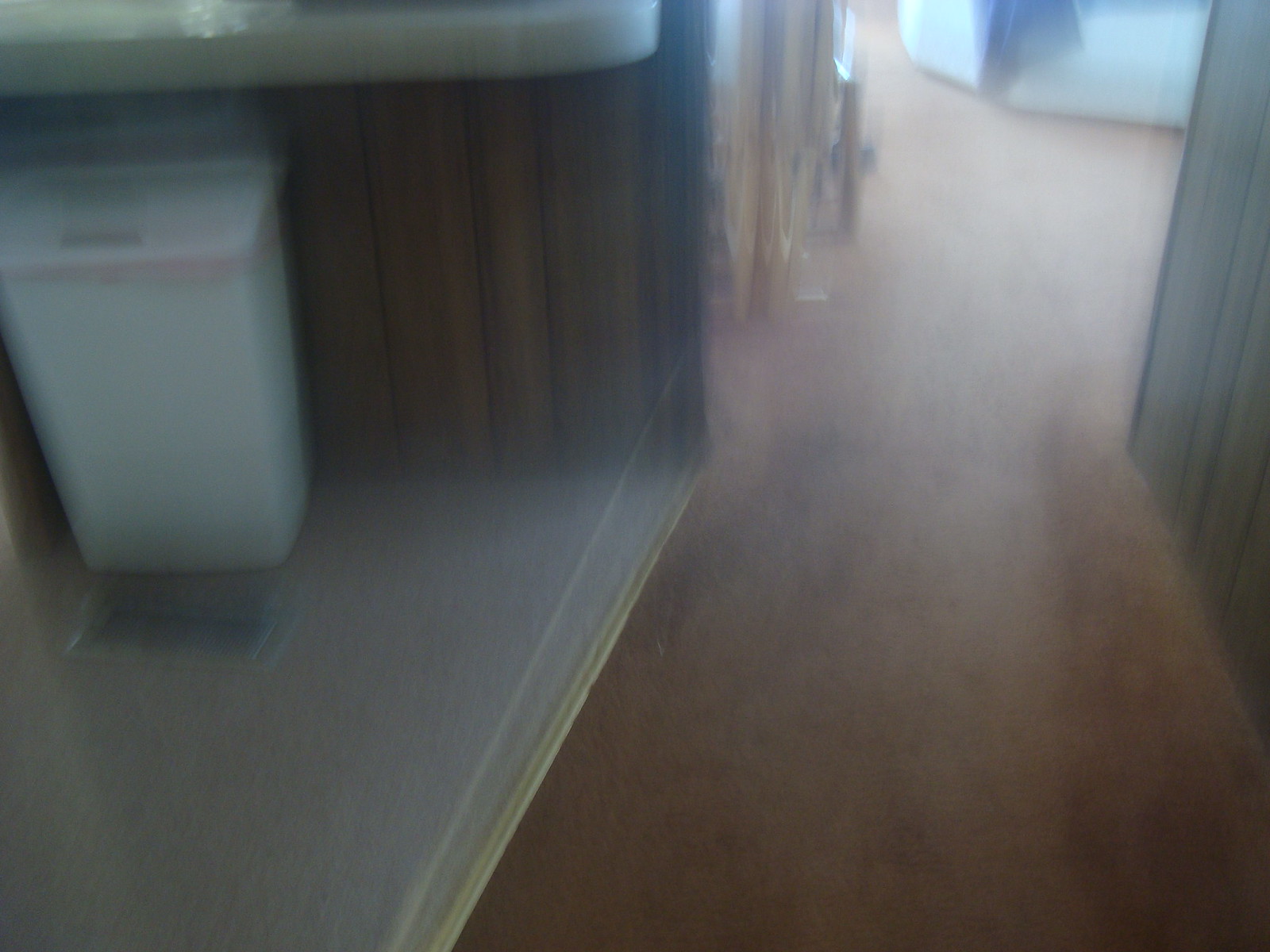The image depicts a blurry hallway that appears to lead into a doctor's office or a similar medical facility. The walls are lined with dated, cheesy 1970s-style fake wood paneling. The floor consists of a painted brown concrete surface. On the left side of the hallway, a white tabletop extends from one of the paneled walls, beneath which stands a white trash can with a pink liner. In front of the trash can, there is a floor vent. In the foreground, a white object, possibly a table, is visible.